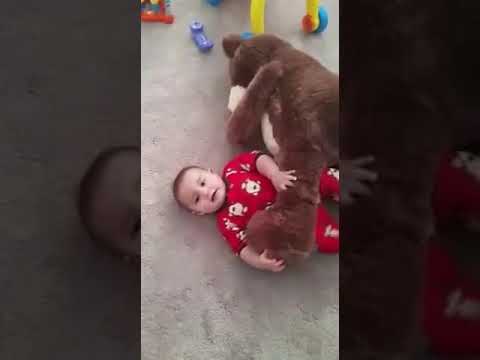This color photograph, captured in portrait orientation amidst a split-screen layout with the sides darkened, showcases a young toddler with dark hair and light skin, smiling directly at the camera. The toddler, likely no more than a year old, is lying on a grayish-beige carpet wearing a red onesie adorned with an indistinct white pattern. This cheerful child is clasping the leg of an oversized brown stuffed bear that lies on its side beside them. The stuffed toy, appearing nearly twice the size of the toddler, has its leg draped across the child's chest. Surrounding the bear are various baby toys including a noticeable purple toy phone and a couple of other colorful items, partially visible atop the bear's body. The vibrant scene exudes a sense of playful innocence and joy, frozen in a moment of childhood bliss.